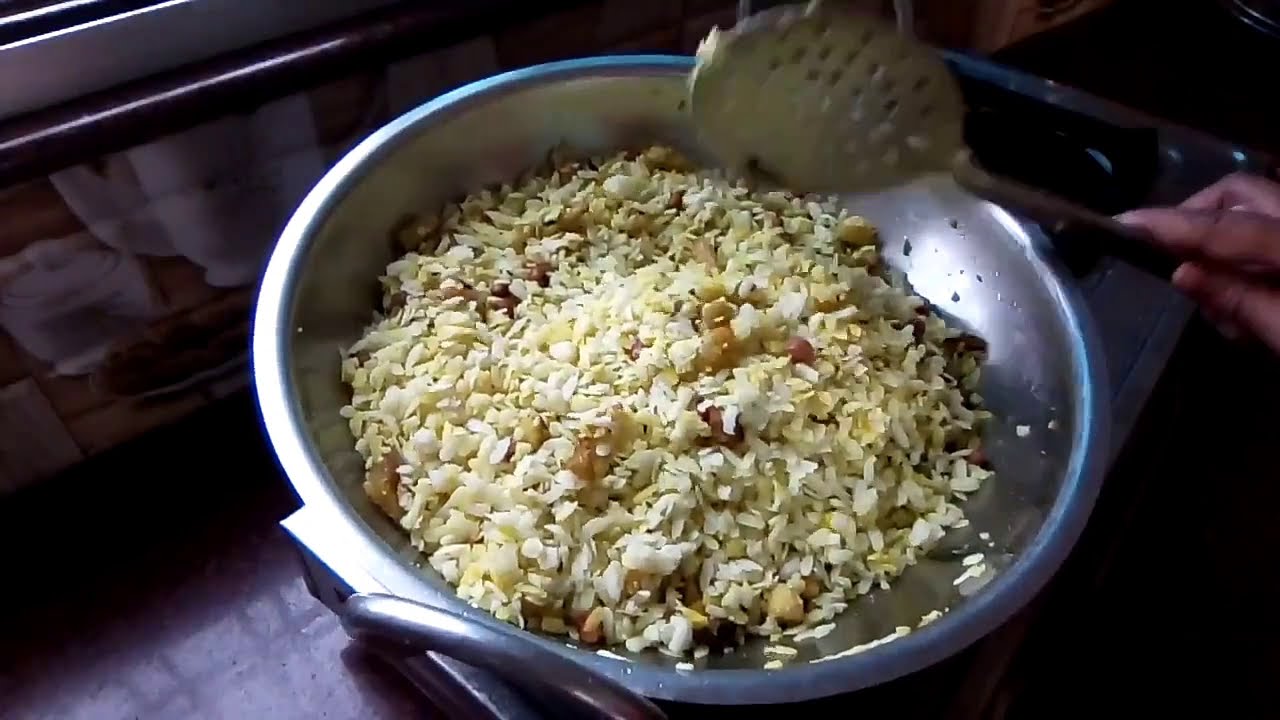The image depicts a large silver bowl with a top handle containing white rice with yellow corn kernels and brown beans, creating a colorful mix. A perforated, circular spatula is partially immersed in the rice, held by a right hand, of which only three fingers are visible – the thumb, index finger, and a bent middle finger. The spatula has a silver handle that transitions to gray near the hand. The bowl sits on a dark surface with shadows and a lighter area underneath. In the background, a wall with horizontal lines and a railing is visible, along with the top outline of a silver rectangle metal tray. Additionally, a box featuring a teacup and sugar bowl can be partly seen, as well as a hint of an appliance, possibly a stove, on the right side.